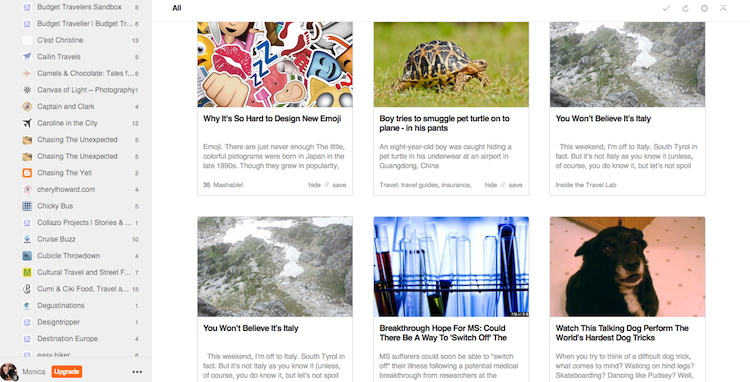The image showcases a webpage with a dual-column layout. On the left side, there is a vertical menu listing various options, including "Budget," "Traveler," "Sandbox," "Bachelors," "Sea," "Earth," "Christine," "Khalid Travels," "Cameras and Chocolates," "Carnival," "Soft Flights," "Photography," "Captain and Clerk," "Curling in the City," "Chasing the Unexpected," "Chasing the 80," "Cherry," "Howard.com," "Cheeky Bus," "Collage of Projects," "Cruise," "Bars," "Cubicle," "Draw Town," "Cultural Travel and Street," "Come and Kid Food," "Castinations," "Design Trip," and "Design Europe." An orange 'Upgrade' button is positioned at the bottom left corner of this menu.

On the right side, the content area features several articles with corresponding images. The first article, titled "Why is it so Hard to Design New Emoji?", raises questions on emoji design. The second article reads "Boy Tried to Smuggle a Pet Turtle onto Plane in His Pants," accompanied by an image of a turtle. The third article, titled "You Won't Believe it: Italy," shows a picture of rocky terrain and is repeated in the bottom left corner with the same headline. The penultimate article titled "Breakthrough Hope for MS: Could There Be a Way to Switch Off?" shows light blue test tubes, while the final article, "Watch This Talking Dog Perform the World's Hardest Dog Trick," features a black dog with brown fur on its chest.